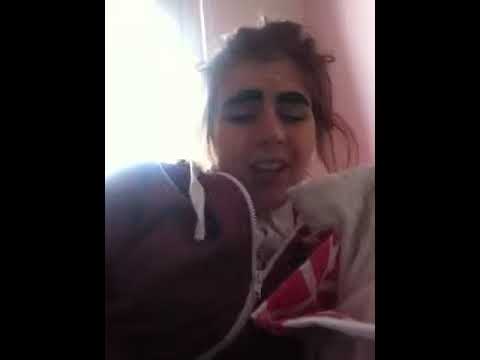The image is a still from a video, capturing a young woman who appears to be in a bedroom. The focal point is her face, which is heavily made up with well-defined eyebrows and striking eyeshadow. Her long, red-dyed hair is somewhat disheveled, tied in a messy ponytail. She is dressed in a burgundy zip-up sweatshirt with a white zipper, and a purple jacket can be seen draped around her. Her mouth is open, and her eyes are closed, suggesting she might be in distress or mid-sentence, possibly screaming or getting ready to speak. She has fair skin and is possibly a college student. The background features a pink-colored wall and a window on the left side, through which bright white sunlight streams in. The room contains various pieces of clothing and a black-colored bicycle on the right side. A white pillow and a red fabric with a white design are also visible in the frame, adding to the cluttered yet intimate setup.